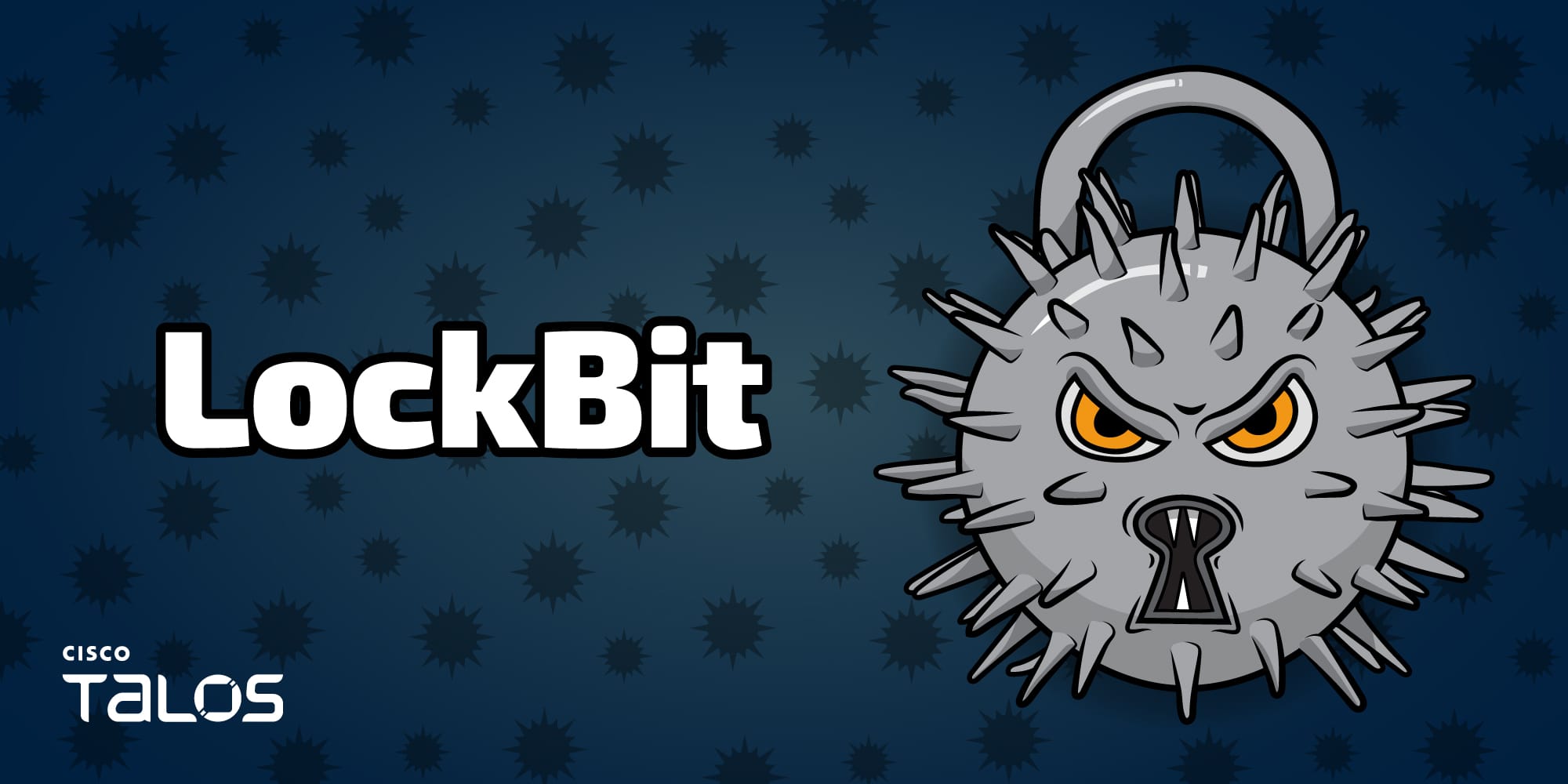This illustrated advertisement for LockBit features a modern, white logo with a capital "L" and "B" against a dark blue background speckled with black, spiky virus-like circles. The lower left corner displays "Cisco Talos" in white font. Dominating the right side is a large, monstrous virus shaped like a lock. This gray, spiky virus has sharp teeth forming a keyhole-like mouth and yellow eyes, topped with an arch resembling a padlock's shackle. The menacing graphic conveys the theme of cybersecurity, suggesting LockBit as a protective, antivirus solution.